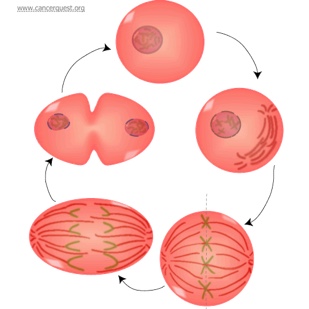The image illustrates the stages of cell growth and division on a white background. At the very top, there is a round pink cell with a darker pink nucleus inside. A black arrow points to the next stage on the right, where the cell, still pink with a now deep red nucleus, begins to develop red filaments. These filaments spread throughout the cell in the subsequent stage, turning it almost entirely pink with gold X-shaped structures appearing down the center. Another arrow leads to a more elongated, oval-shaped cell where the red filaments are spread to both sides, and the cell seems to be pulling apart. In the final stage, the cell divides into two separate egg-shaped cells, each with a dark red nucleus, stretched apart with white V-shapes cutting into the center, indicating the completion of cell division. The top left corner of the image contains the small grey text: www.cancerquest.org.